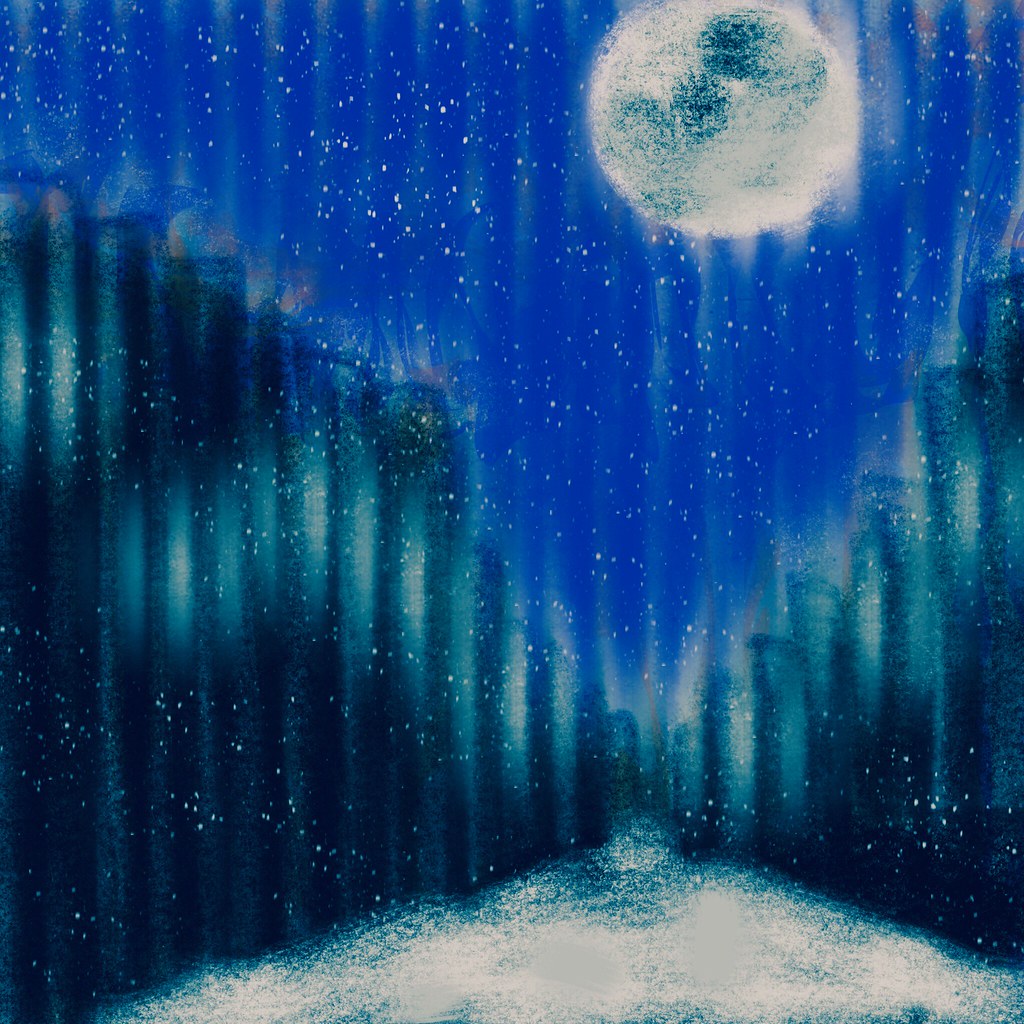The image is a color illustration with a surrealistic and abstract style, making it challenging to determine the precise medium—whether hand-drawn and colored, painted, or digitally created. Dominating the top right corner is an oversized, somewhat inaccurate representation of a moon, featuring greenish-blue patches where craters would traditionally be. The sky, depicted in various shades of blue, is sprinkled with white specks symbolizing stars, intersected by vertical white streaks that give the appearance of light beams. These vertical elements extend throughout the composition, creating a consistent linear motif.

In the foreground, a path or canal stretches away from the viewer, its width narrowing towards the horizon. This path shares the moon's color palette, characterized by a light off-white cream interspersed with bluish-greenish turquoise tints, particularly pronounced as it recedes. Flanking this pathway on either side are unidentified tall structures, resembling girders or rods, primarily dark blue with lighter blue, almost glowing, accents. These structures also emit upward streaks of blue, reinforcing the vertical line theme.

The overall scene exudes a rippling effect, as though the entire image is gently undulating, contributing to its dreamlike quality. There are no signs of life—no people, animals, plants, or any other objects—just the ethereal interplay of color and form creating a serene, otherworldly landscape.